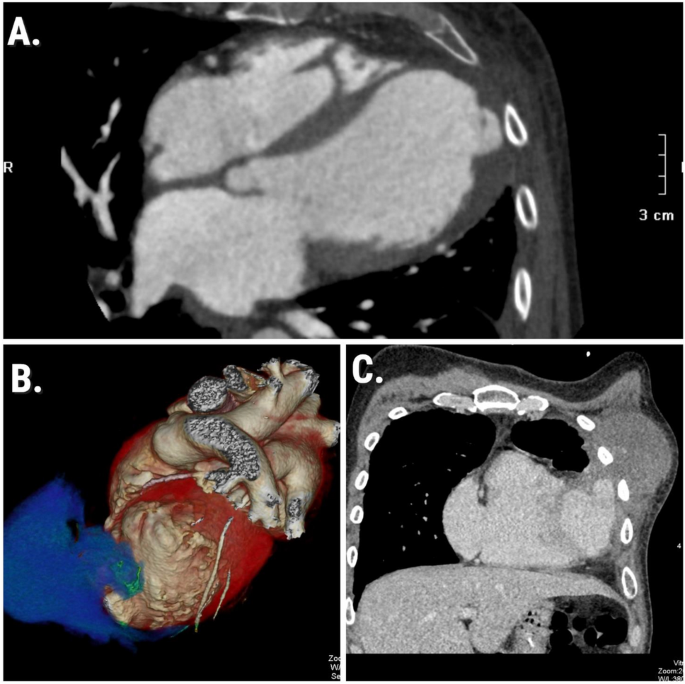This composite image features three panels labeled A, B, and C, arranged in a square format with the rectangular image A at the top and the square images B and C below it. Each panel appears somewhat like a scan or x-ray, depicting different anatomical views and elements, and the entire background is black.

Panel A is a black-and-white image that resembles an x-ray or ultrasound, showing a large gray blob divided into several smaller white blobs within it. Along the right-hand side of this panel, there are lines indicating a scale labeled "3CM." The image evokes the appearance of internal body structures, possibly showing multiple entities within one organ.

Panel B, located in the bottom left, diverges from A by being in color. It portrays an organ that resembles a heart, distinguished by its detailed depiction of tubes, veins, and arteries. The organ displays a gradient of colors from blue at the bottom to white and red, with gold elements visible underneath. This panel provides a more intricate and vivid view compared to the monochrome details of panel A.

Panel C, like A, is in black and white and seems to display another organ encapsulated by the same distinctive metal belt seen in panel A. This panel includes approximately 15 circled areas marked out on the organ, along with white specks scattered throughout. The gray border encasing the organ is annotated with various white marks, as if highlighting specific points of interest.

Overall, the image presents a detailed medical or anatomical depiction across three distinct but related scans, with remarkable emphasis on organ structure, scale indication, and color variation to distinguish different types and levels of detail.